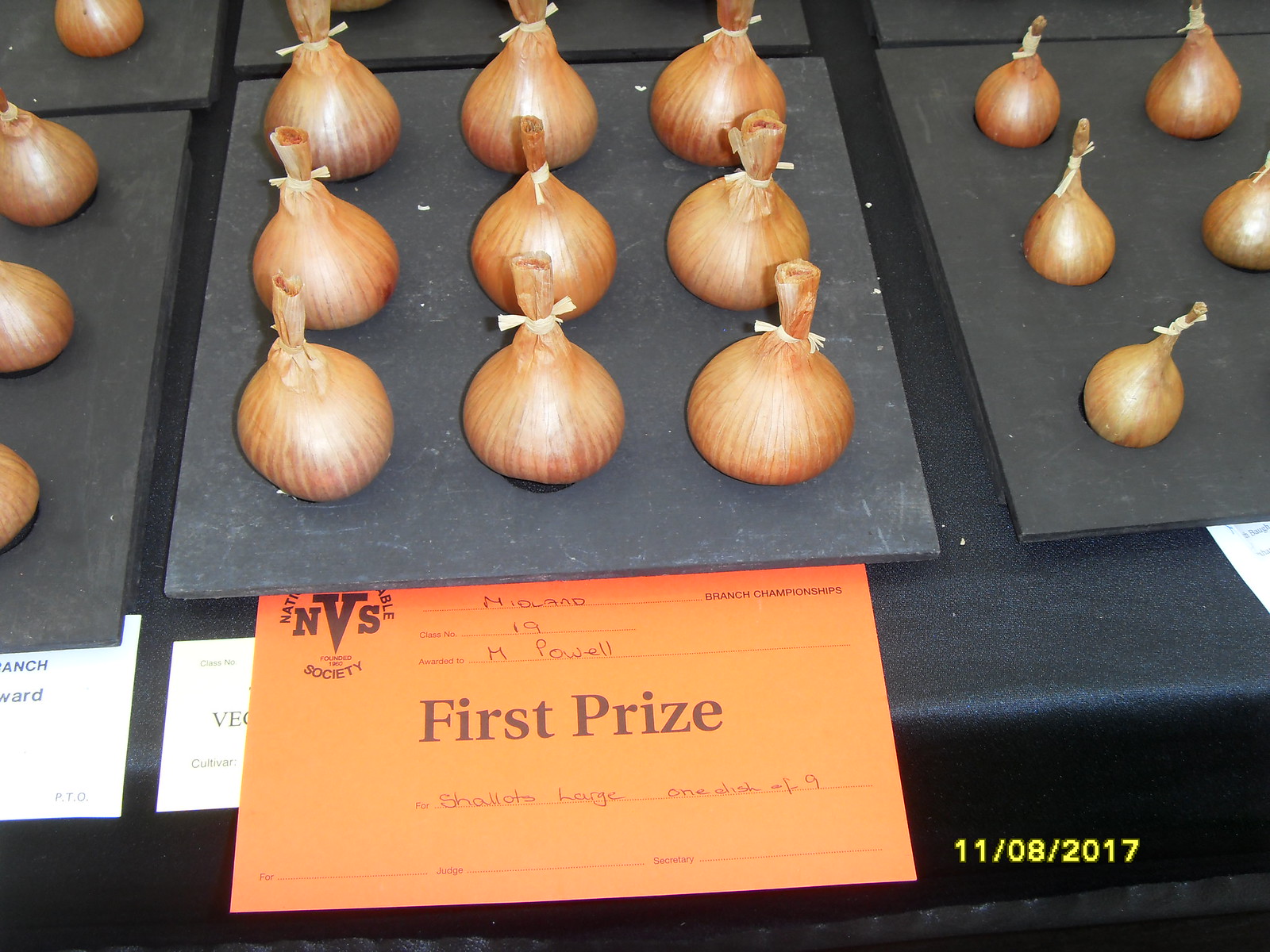In this photograph dated 11-08-2017, a meticulously arranged display of brown shallots is showcased, suggesting participation in a competitive event. The central focus is on a black, matte square board, perfectly aligned with nine shallots arranged in three rows and three columns. Surrounding this central board are partial views of additional similar square boards, each displaying its own grid of nine shallots. Beneath the main board, there is an orange poster with the prominent black text "First Prize," indicating a successful entry. The poster details Midland 19 M. Powell of the Envia Society as the winning participant for the "Shallots Large" category. This elegant arrangement suggests a formal event where presentation and uniformity were key evaluation criteria.